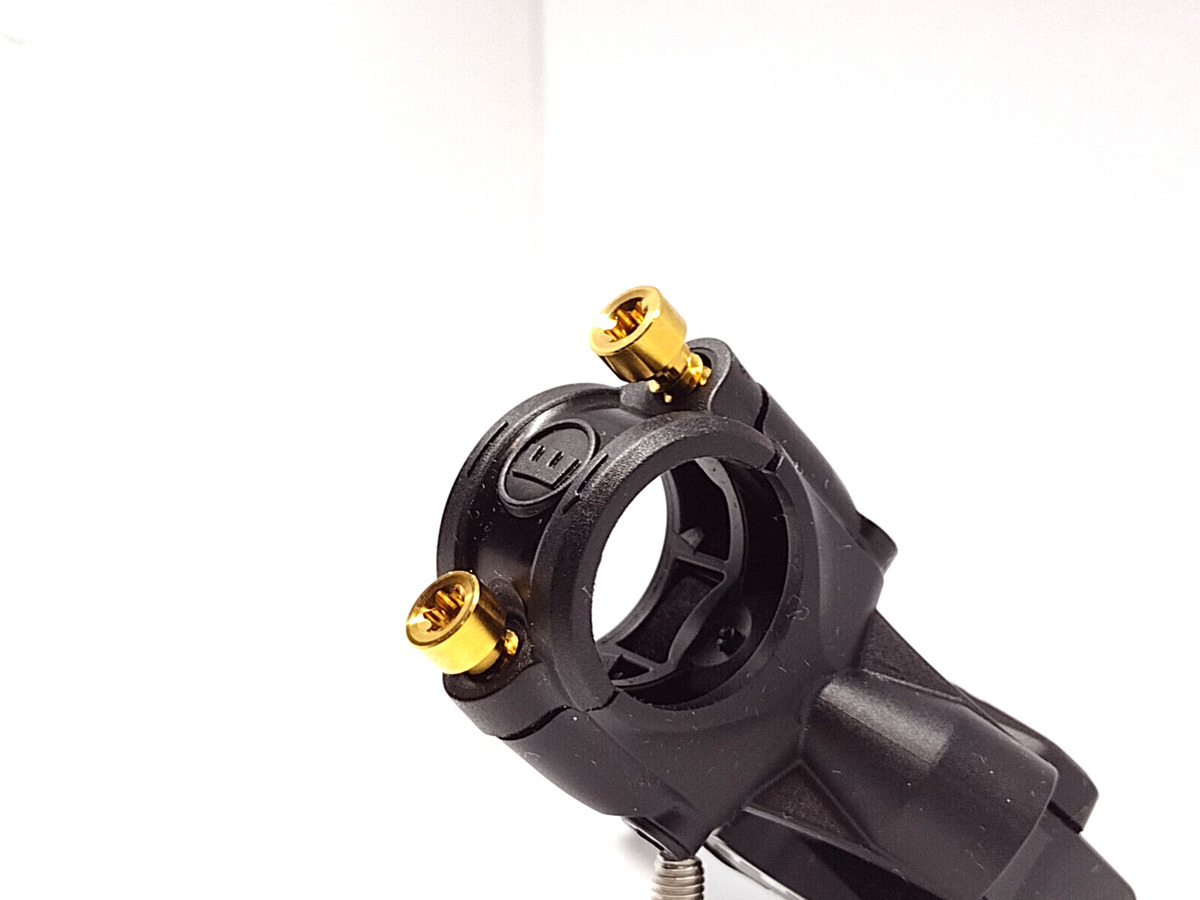This image showcases a black plastic tool or connector, possibly a hose clamp, placed against a white background. The tool features a handle that extends downward, though the image cuts off before revealing its full length. At the top of the handle, there is a circular opening, allowing visibility through the center, and on either side of this circle, two fixtures with gold or brass hex bolts are embedded into the black plastic. These bolts appear to be designed for attaching or screwing in additional components. Prominently displayed at the top of the black plastic piece is a raised circle with the letter 'E' inscribed on it, accompanied by a few indentations around the letter. Additionally, there is a single gray metal screw situated at the bottom, completing the overall structure of this visually distinctive tool.